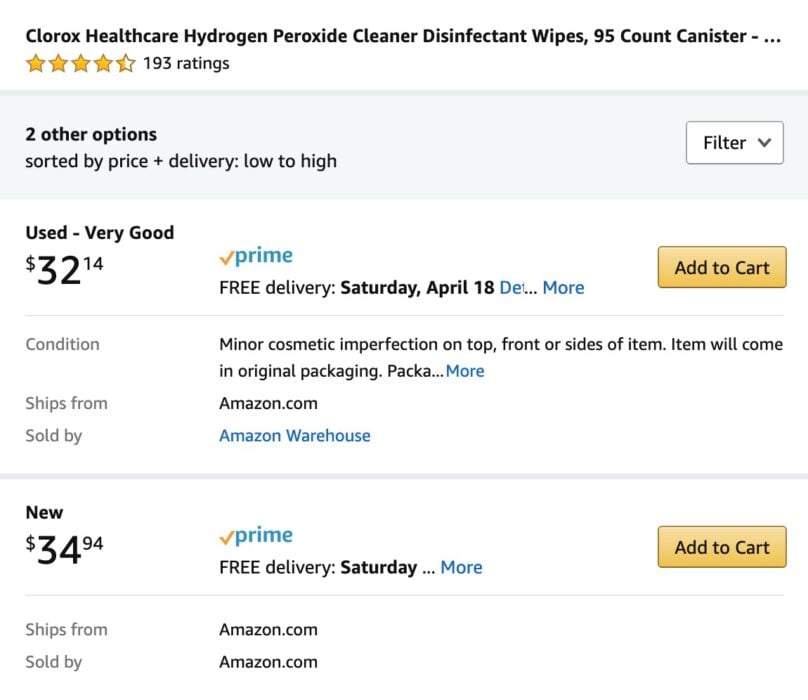This image is a screenshot from Amazon's website showcasing the product, "Clorox Healthcare Hydrogen Peroxide Cleaner Disinfectant Wipes, 95 Count Canister." At the top, the product name is clearly displayed. It has garnered 193 ratings, averaging around 4.5 out of 5 stars, indicated by four fully filled stars and a half-filled fifth star.

Beneath the product title, there are sorting and filtering options, currently set to arrange by price and delivery from low to high. A drop-down menu provides additional sorting options. 

The first visible product listing is for a used item in "very good" condition priced at $32.14, available through Amazon Prime with free delivery on Saturday, April 18th. The condition note mentions minor cosmetic imperfections on the top, front, or sides of the item, which will arrive in its original packaging. This item is sold by Amazon Warehouse. An orange "Add to Cart" button is prominently displayed.

The second listing is for a new item priced at $34.94, also available through Amazon Prime with free delivery on Saturday. This item is sold by Amazon.com. A yellow "Add to Cart" button is provided.

The listing may seem expensive for a 95-count canister, which might be indicative of the time during the early stages of the COVID-19 pandemic when disinfectant products were in high demand and often difficult to find.